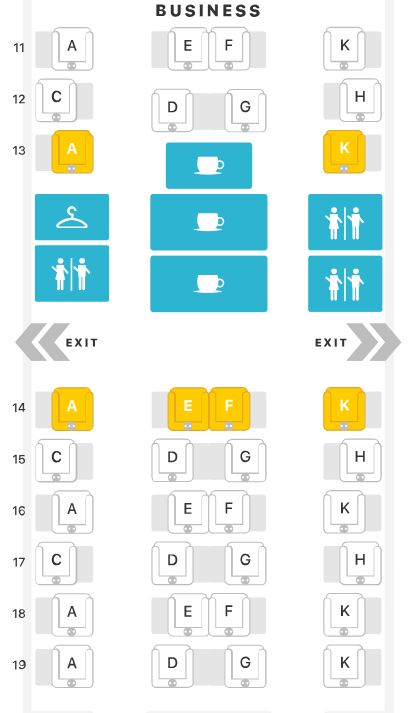The image appears to be a schematic representation of a business website, featuring an organized business chart. The layout is framed with a light gold bar running vertically along both the left and right sides. 

At the top center, the word "Business" is prominently displayed in large, bold black letters. Along the left edge of the chart, numbers 11, 12, and 13 are sequentially listed. The chart contains several labeled sections: small white squares marked with the letters A, E, F, and K, as well as additional white squares labeled C, D, G, and H.

Two yellow squares within the chart are labeled A and K. Nestled between these is a blue square depicting a teacup icon. Beneath this square, there are two larger blue squares, each also featuring a teacup symbol. 

To the left of the blue teacup square, there is an icon of a hanger, and directly below this, a blue square displaying male and female images, seemingly waving. Additional icons to the right of the teacup square include male and female figures, with another set of male-and-female images beneath them.

Both the left and right sides of the chart are marked with exit signs. Grey arrows are present within the layout, likely indicating directions or flow within the chart. 

Further down the left side, numbers 14 through 19 are sequentially listed. In section 14, there are gold blocks labeled A, E, F, and K. The remainder of the sections (15 through 19) continue the pattern with different letters placed in various configurations.

Overall, this structured and color-coded chart appears to be a detailed overview of the business website layout or navigation map, showcasing various sections and their interconnected parts.